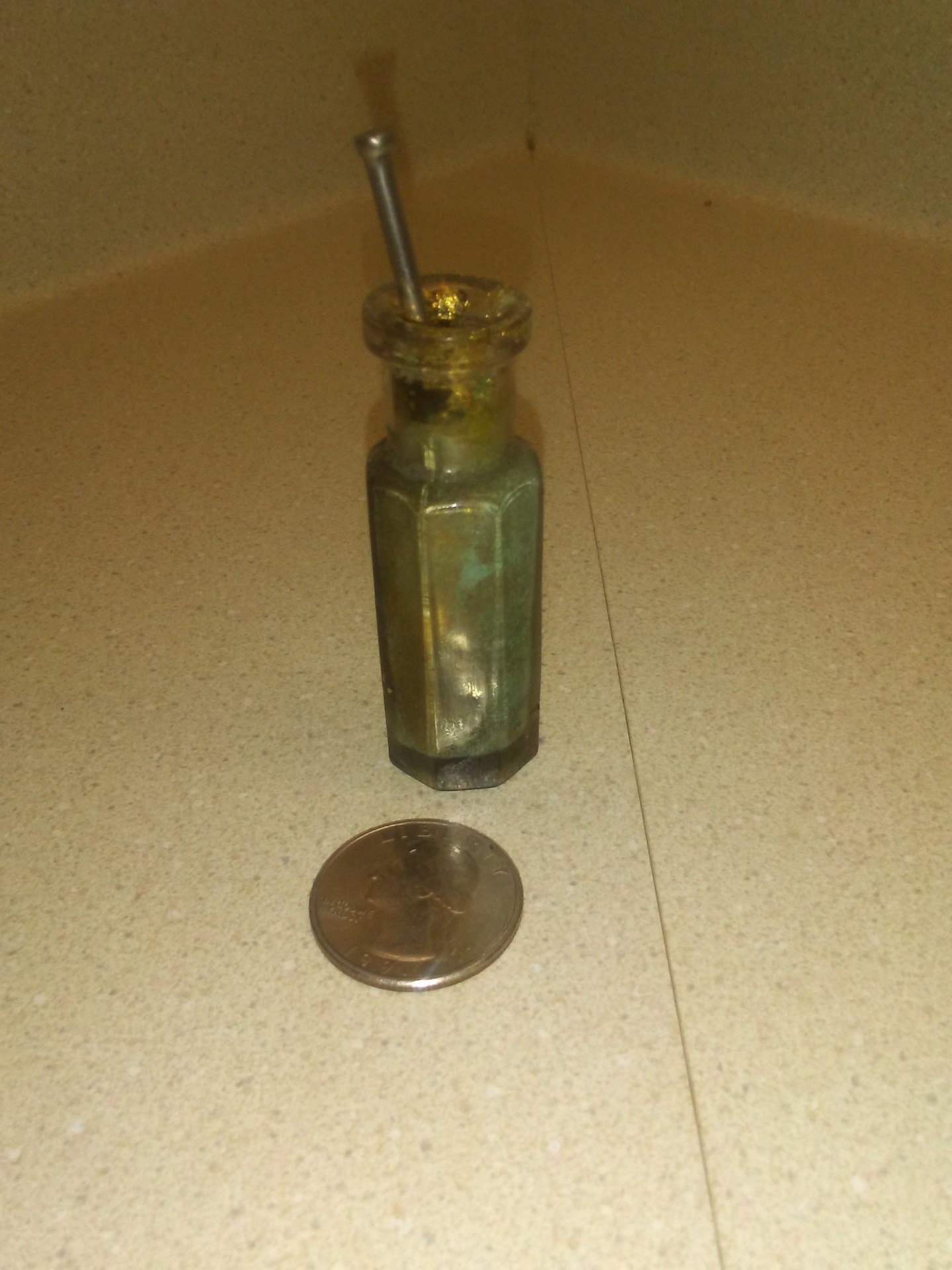The image depicts a vertically-oriented color photograph, capturing a small, dark green glass bottle with angular, cylindrical sides, situated on a speckled countertop with gold and brown hues. The bottle, which has a notably thick rim at the top, contains a metal rod protruding several inches above it, resembling a nail or a cylinder with a rounded end. For size reference, an American quarter lies flat on the countertop in front of the bottle, demonstrating the bottle's very small scale. The scene, poorly lit with dim lighting, is set in a kitchen, evidenced by the countertop's seam running down the middle and the tile floor's single visible line extending towards the back where two walls meet at a corner. The bottle's greenish color appears opaque and slightly metallic or shiny, further adding to the image's cryptic nature and dim ambiance.